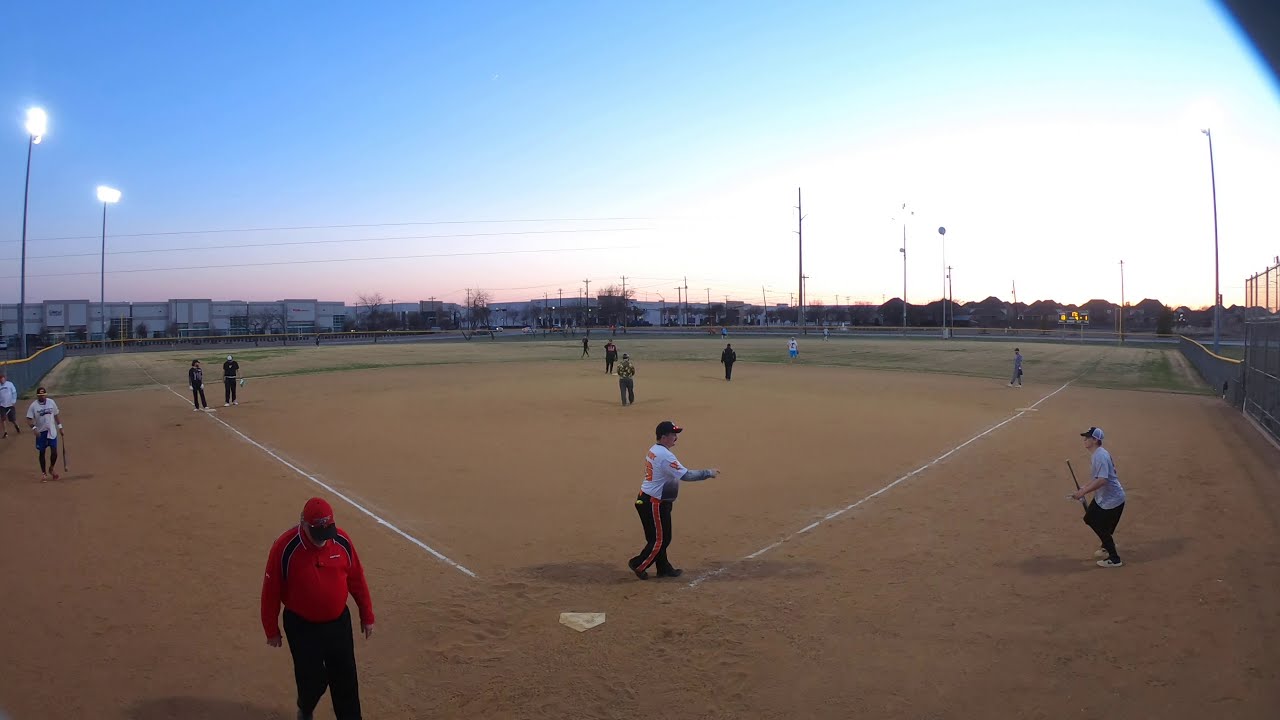In this photograph captured at a baseball field, the scene is set near twilight, likely either at sunrise or sunset, given the dim light and illuminated tall outdoor lights. The focal point near home plate shows a coach or possibly a referee in black pants, a long-sleeved red shirt, and a matching red cap, walking with his head down, likely between plays. The field is a smooth, beige dirt expanse with white lines denoting the bases, one of which is visible in a corner of the image where a large boy stands sideways near it. 

In the background, suburban houses with a few illuminated lights and some bushes and trees suggest a rural or suburban setting beyond the field's fence. The players on the field are mostly dressed in black sweatshirts over their uniforms, indicating a cool evening, with a mix of white jerseys with orange lettering. A catcher, identifiable by his gear, appears to be addressing a player holding a bat halfway down the first baseline, possibly giving instructions. There are twelve players scattered across the field, some preparing for what seems to be a night game, each engaged in different activities.

The quality of the photograph is poor and blurry, making it difficult to distinguish many figures apart from the coach, the catcher, and the player with the bat. The sky above shows the fading light of dusk, framing this quiet but anticipatory scene of pre-game preparations.